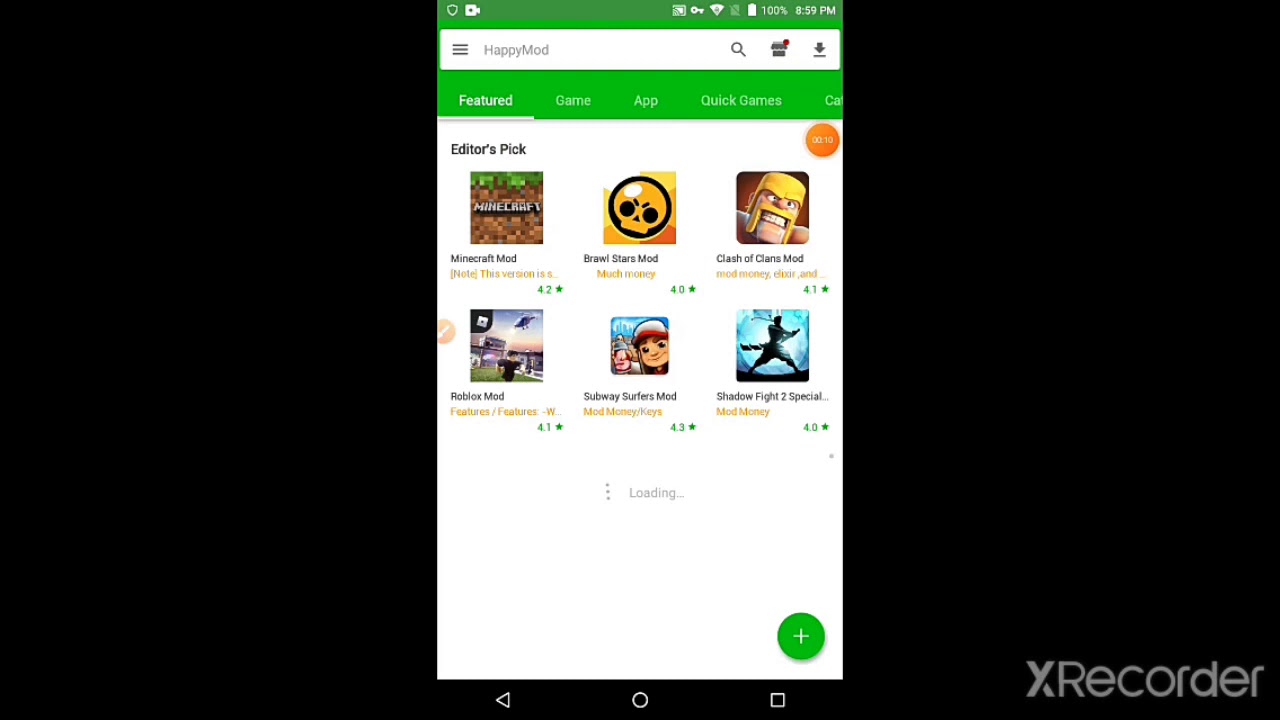The image showcases a black background screen with the X Recorder application interface on the right side in gray. At the bottom of the screen, there are three white-outlined symbols: a triangle on the left, a circle in the middle, and a square on the right. The screen features a green banner at the top indicating the time as 8:59 p.m. on the right side, along with a fully charged, 100% battery symbol and a Wi-Fi icon. To the left of the banner, there is a white camera icon. Below this, the screen shows three horizontal lines labeled "Happy Mod" accompanied by a magnifying glass symbol for the search function. There's also an icon that resembles a house, likely representing the home button, followed by a download arrow symbol.

Further down, a green bar spans across the screen with white text that reads, "Featured Game App, Quick Games," though the text appears to be cut off. Below this green bar is a white background with black text that reads, "Editor's Pick," followed by various app images along with their ratings. The first is an image for Minecraft, labeled "Minecraft Mods," with a rating of 4.2 stars. 

Next is an image for "Brawl Stars Mod," rated at 4.0 stars, followed by "Clash of Clans Mod,” which includes an orange circle with some unintelligible white text, and depicts an image of a character with a yellow head that appears to be angry. 

The subsequent line displays "Roblox Mod," with a 4.1 rating, followed by “Subway Surfers Mod,” showing an image of a little girl and boasting a 4.2 rating. The final displayed app is "Shadow Fight 2 Special," showing what possibly depicts a person walking in moonlight, having a rating of 4.0 stars. At these app images' base are three vertical dots representing a loading indicator in gray, with some yellow writing that is indecipherable under each image.